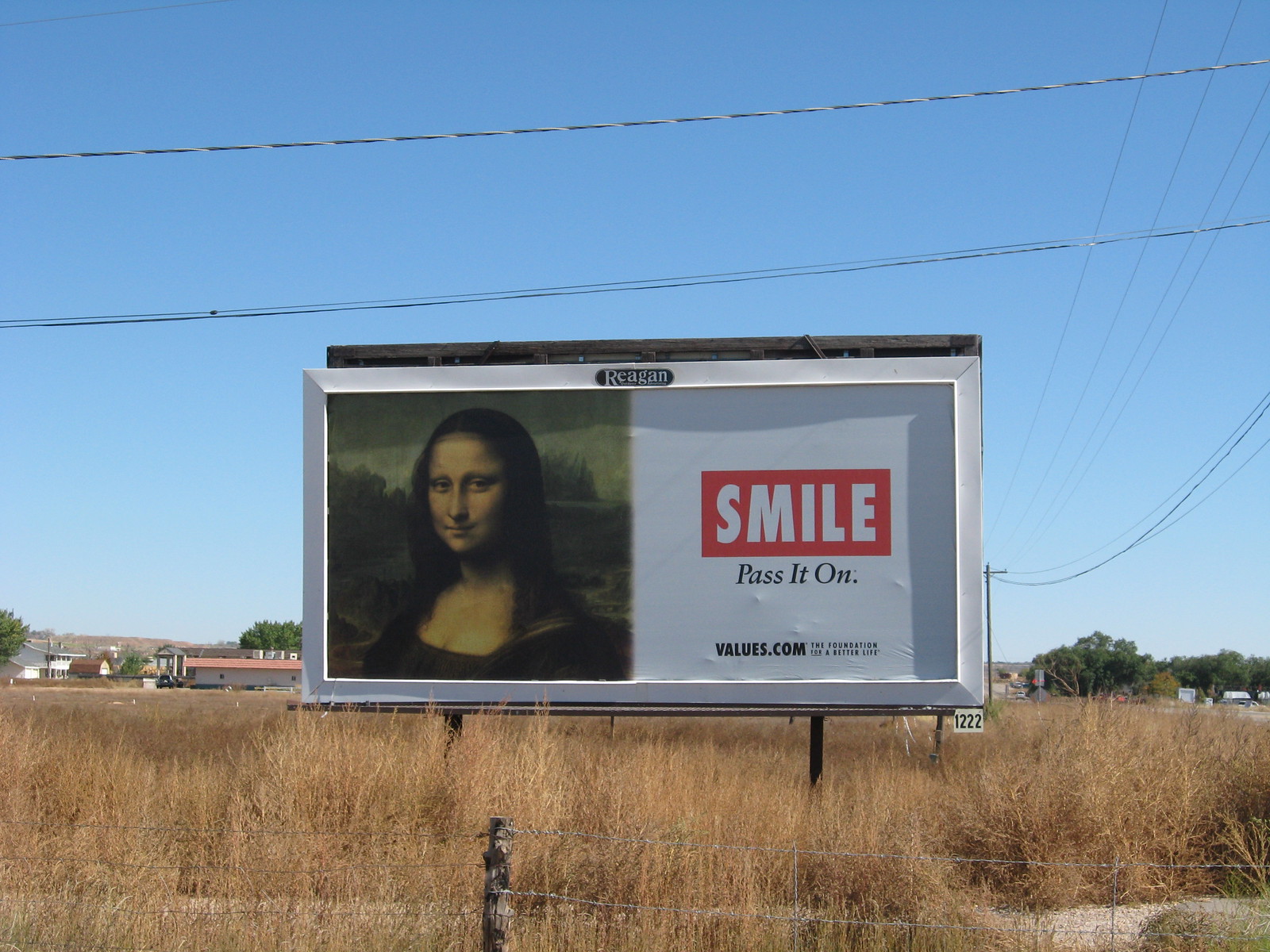A vibrant color photograph captures a rural billboard set against a pristine blue sky devoid of clouds. Suspended above the billboard, an intricate web of utility wires crisscrosses the scene. A particularly notable wire, braided with an aluminum strand, stands out among the array of black cables and a network of horizontal wires stretching into the distance and affixed to a telephone pole.

The landscape around the billboard indicates a rural setting, characterized by tall, browned shrubs and grasses, likely signifying the autumn season. In the immediate foreground, a rustic wire fence supported by weathered wooden posts runs parallel to the scene.

The billboard, framed in a white mitered border, prominently features the number “1222” at its bottom right corner. At the top of the billboard, an oblong black plaque with the word “Reagan” indicates the company responsible for the advertising space. Dominating the left side of the billboard is the iconic image of the Mona Lisa. To the right, a stark white background is interrupted by a bold red rectangular text box containing the word “SMILE” in large, white capital letters. Beneath it, the message continues with “PASS IT ON,” followed by a period. This motivational slogan is sponsored by VALUES.COM, although finer details below the text are unreadable.

In the idyllic background, low rolling hills provide a gentle horizon, dotted with what appears to be low houses or farmsteads and mature shade trees scattered on both the left and right sides, adding to the serene rural charm of the photograph.